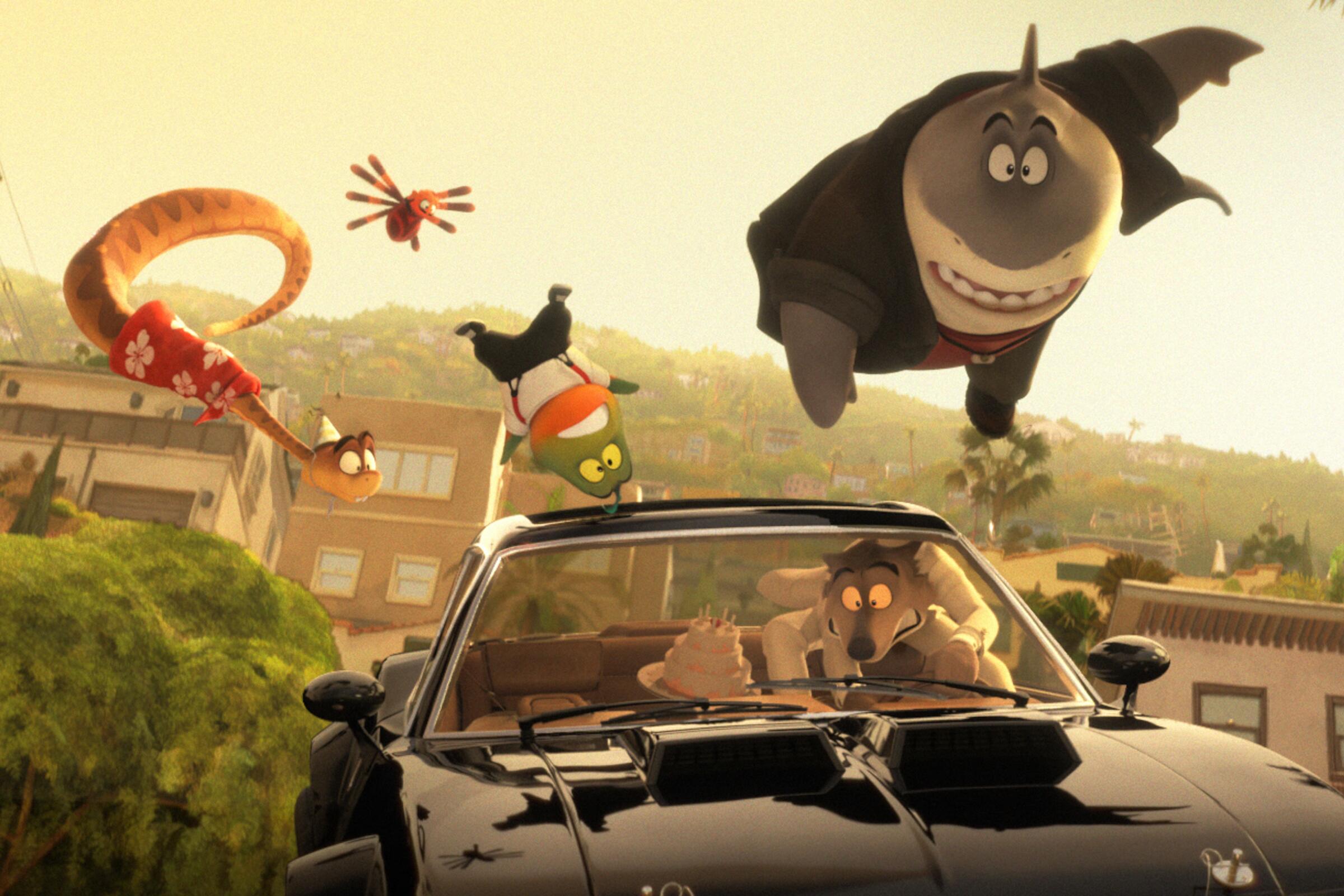This is a highly detailed animated scene, evocative of a Pixar movie, featuring a lifelike black sports car convertible driven by a panicked, cartoon wolf with yellow eyes and a black nose, distinguished by its light tannish-brown fur. The wolf, gripping the steering wheel anxiously, has a three-tier wedding cake placed either on the dashboard or the backseat of the car. Surrounding the car are additional animated animal characters caught in mid-air above it. To the left, a snake wearing a red and white Hawaiian shirt can be seen, followed by a spider with its eight legs sprawled. Above the car flies an upside-down frog dressed in suspenders, a white shirt, and black pants. A sizable shark in a dark green, open button-down shirt is also suspended in the sky. The background features a slightly blurred environment consisting of hills, buildings, and greenery, all bathed in what could be the golden light of sunset. The scene is whimsical, capturing a moment of chaotic hilarity.